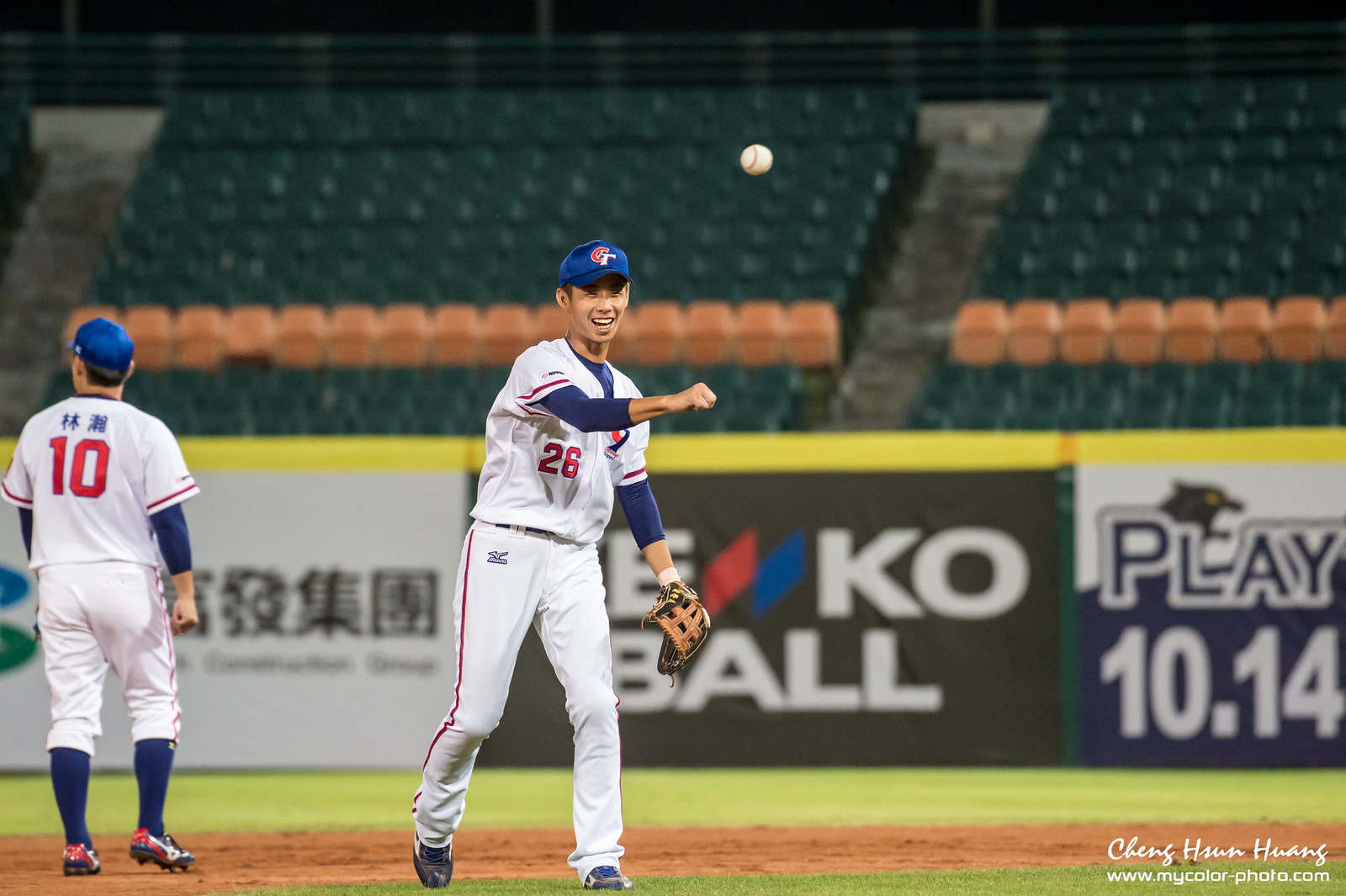The photograph captures a vibrant moment on a neatly manicured baseball field, characterized by its short green grass and tan-colored dirt. In the bottom right corner of the image, the watermark reads "Chang Han Horns, mycolor-photo.com." Two baseball players are prominently featured, both sporting white jerseys adorned with Asian characters and red numbers. The player on the left, positioned at the corner of the frame, has the number 10 on his back and is dressed in white pants with red side stripes, long blue socks, and red-and-white cleats. The player on the right, facing forward and smiling as he completes a pitch, has a red number 26 on the front of his jersey. The baseball he has just thrown is visible mid-air in the top center of the photograph. Both players wear blue hats, and their uniforms evoke the color palette reminiscent of the Los Angeles Dodgers. The scene suggests a youthful, possibly non-professional game, given the distinctive Asian script on their jerseys.